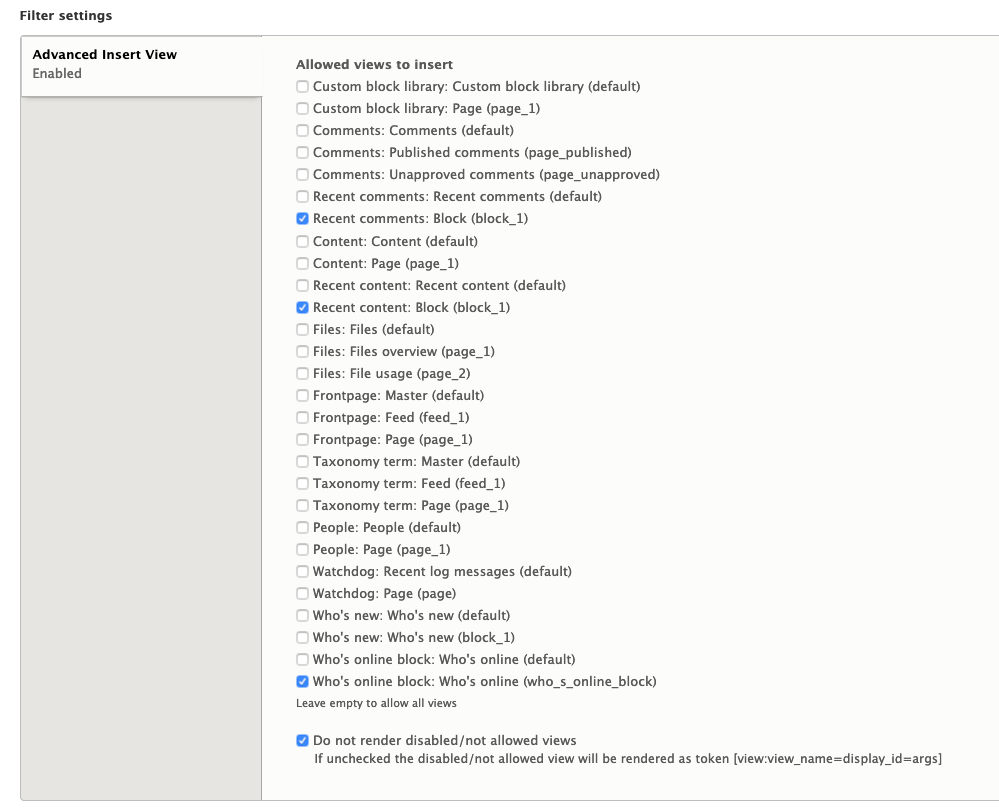This image is a cropped screenshot taken from the admin panel of a website's filter settings section. At the top left, the header "Filter Settings" is displayed in small black letters. Directly beneath this header, the term "Advanced Insert View" is written in bold, yet very small black letters within a large grey box. Following this, the word "Enabled" appears in small black letters.

Adjacent to the grey box on the right, there is a light grey panel that extends from the center left of the page to the far right. At the top of this panel, the heading "Allowed Views to Insert" is prominently featured in bold text. Below this heading, there is an option labeled "Custom Block Library" accompanied by a checkbox on its left. The entry "Custom Block Library Default" follows this, but it is not checked. Further down, "Custom Block Library Page, Page 1" is also listed but remains unchecked. This pattern continues vertically down the page.

Out of the listed items, only a few checkboxes are ticked, indicating enabled options: "Recent Comments Block, Block 1," "Recent Content Block, Block 1," and "Who's Online Block, Who's Online Block." Below the list, a message reads "Leave empty to allow all views." Finally, at the very bottom, there is a note: "Do not render disabled not allowed views. If unchecked, the disabled not allowed view will be rendered as a token." The corresponding checkbox for this option is also checked.